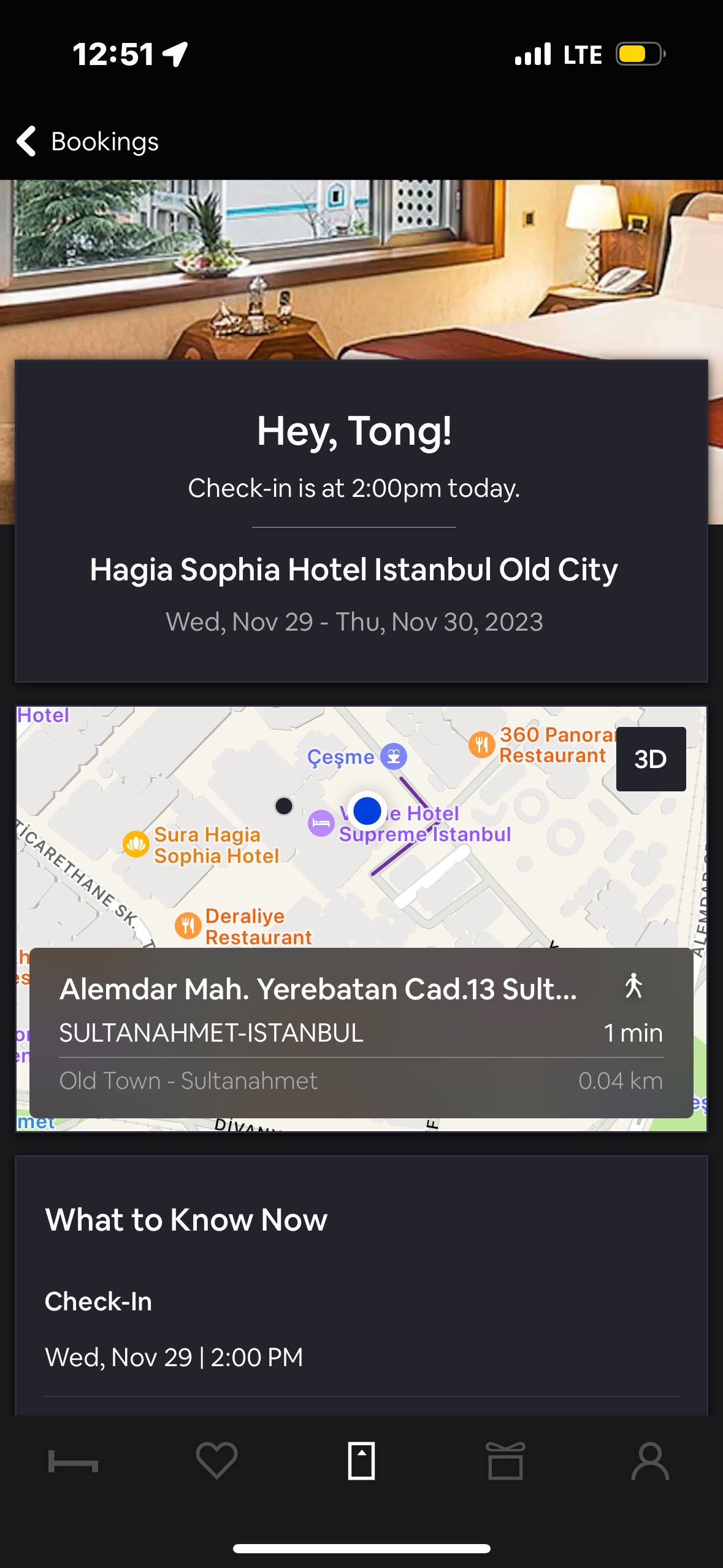A screen capture from a mobile device displays a predominantly dark gray interface. At the top portion of the screen, there is a partially obscured image depicting an interior room. The room has cream-colored walls and features an open window through which an exterior building is visible, characterized by its gray facade with a prominent blue stripe. A small green potted plant adorns the windowsill, adding a touch of nature to the scene. Inside the room, a bed with white sheets is noticeable, along with a brown strip at its base. The window frame is also visible within the room. The lower portion of the screen showcases a map application, above which white text reads: "Hey Tong, check-in is at 2 p.m. today Hagia Sophia Hotel Istanbul Old City."